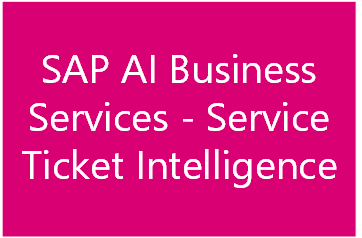In this vibrant and eye-catching image, a hot pink rectangle is displayed in a landscape orientation. The rectangle features three centered lines of white text, all in Sans Serif font, potentially Arial. The top line reads "SAP AI Business" with "SAP" and "AI" in uppercase letters and "Business" in title case. The second line states "Services-Service," and the third line reads "Ticket Intelligence." All text is aligned along the center, giving the layout a balanced appearance while ensuring the edges of the text do not align.